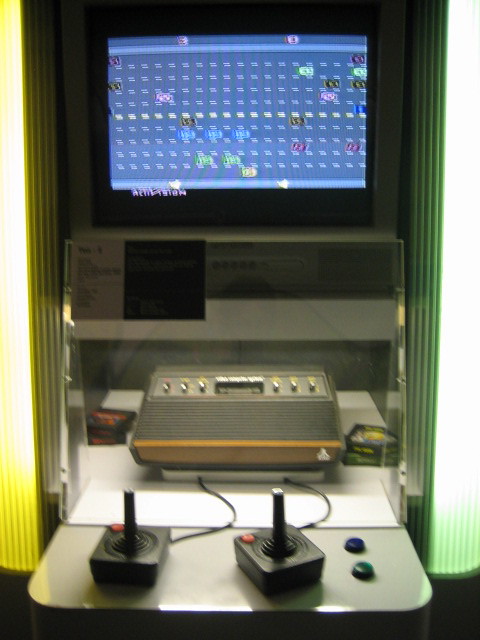This is a color photograph depicting a vintage arcade game console likely from the 1970s or 1980s. The image captures the old-school charm with distinct yellow and blue panels flanking the left and right edges of the machine. At the top of the console, a blue screen is visible, dotted with numerous small perforations. Tiny characters in colors of blue, pink, and green are seen navigating across what resembles a network of roads on the screen. Below this, the game screen is housed within a robust metal casing.

Beneath the metal casing sits a rectangular console featuring metallic knobs on its upper section, transitioning to a wooden finish towards the bottom, adding a vintage aesthetic. This part of the console appears to have grey lines running through it, potentially indicating a sound system or simple design lines. At the base of the console, two simplistic game controllers are placed on a metallic surface. These black controllers are equipped with sticks and feature a red circle in the upper left corner of each. Additionally, two round knobs are situated just to the right of the controllers on the metallic surface, completing the nostalgic setup.